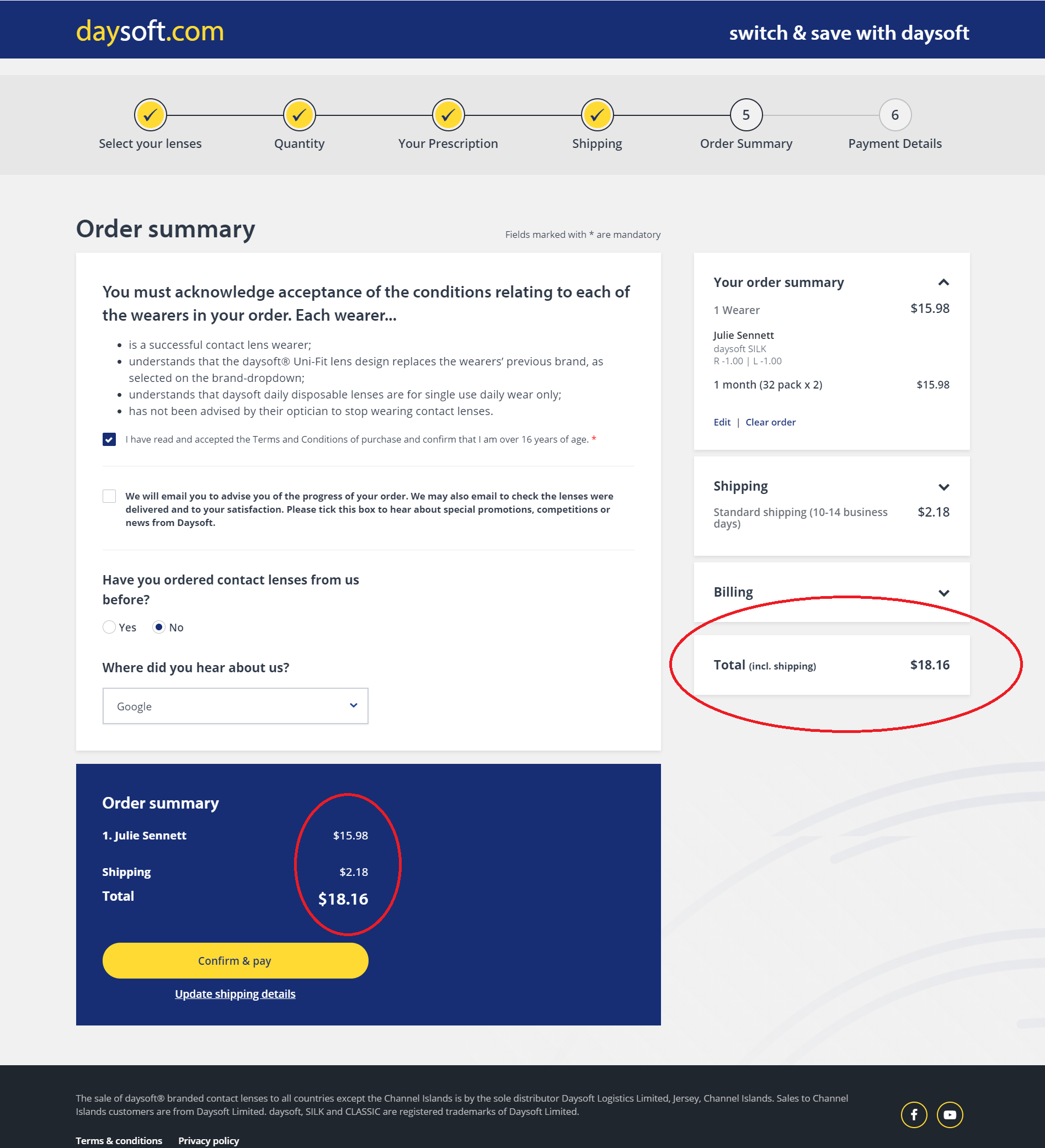This image showcases an order confirmation page from the e-commerce website Daysoft.com.

At the top of the page, a navigation bar displays the brand's name, "Daysoft.com," alongside a promotional tagline, "Switch and Save with Daysoft," on the right. Below this, a multi-step timeline visually guides the user through the order process. The steps include:

1. Select Your Lenses
2. Quantity
3. Your Prescription
4. Shipping
5. Order Summary
6. Payment Details

The first four steps are visually highlighted in yellow and each has a check mark, indicating their completion. The last two steps, "Order Summary" and "Payment Details," remain unchecked, suggesting that the order is nearly complete but not yet finalized.

In the middle section of the page, a detailed list of terms and conditions is presented. To the right, an order summary details specific information such as the wearer's identity, the type and quantity of contact lenses ordered, the shipping charge, and the total billing amount.

At the bottom of the page, there is a breakdown of the total price, including shipping. This section also features a prominent "Confirm and Pay" button highlighted in yellow, inviting the user to finalize the purchase. Next to this, a secondary button labeled "Update Shipping Details" provides an option to modify shipping information.

The footer at the very bottom includes links to important legal documents such as the terms and conditions, privacy policy, and a disclaimer, as well as icons linking to various social media sites.